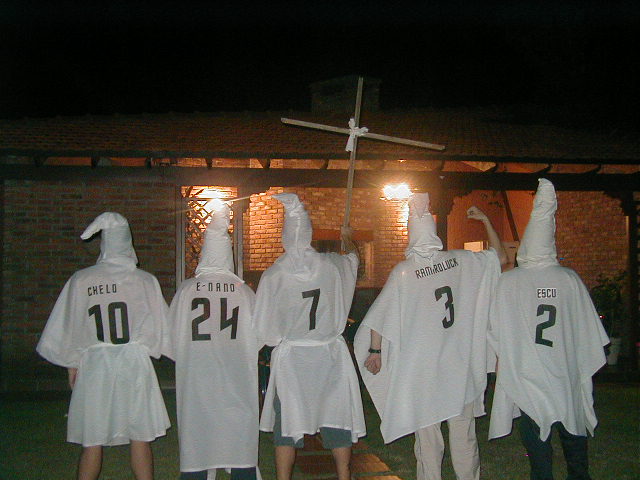This image shows a highly offensive and inappropriate scene of five individuals dressed in Ku Klux Klan robes, which have been altered to resemble soccer jerseys. The white robes feature numbers and nicknames such as Cello 10, Inano 24, and Ramrolik 3, while one individual, number 7, chose not to display a name. These individuals are positioned in front of a cross, with some posing with their hands raised in apparent mockery. The backdrop suggests it is nighttime, and they stand in front of a house. The image conveys a disturbing attempt at humor that evokes hate and insensitivity, reflecting poorly on those involved.